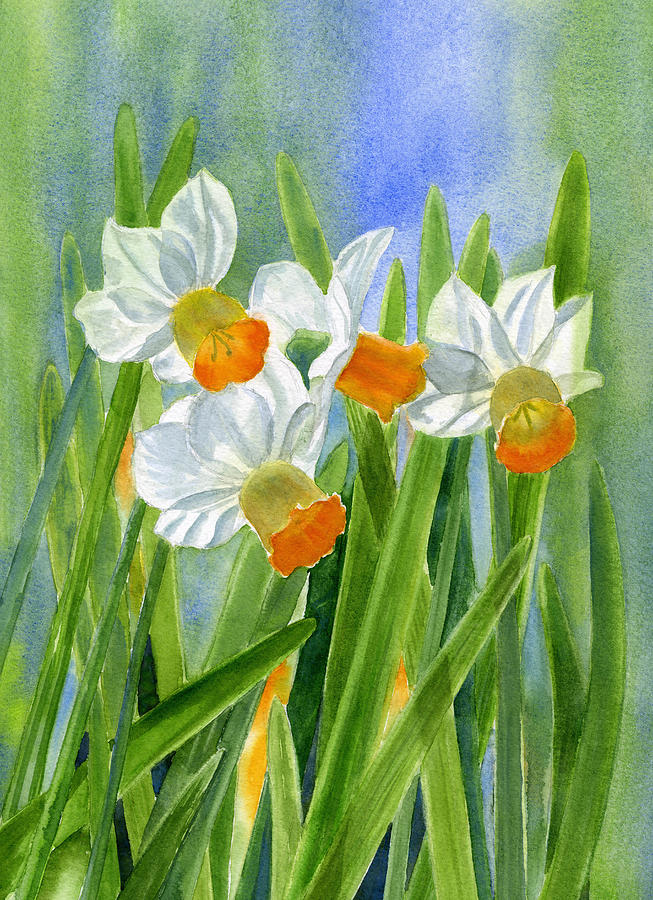This detailed illustration presents a vibrant watercolor painting of flowers, potentially daffodils, showcasing an array of white petals with golden-orange centers. The flowers, four in total, bloom prominently two-thirds from the bottom of the piece, amid long, dark green stems and fronds. The background enhances the composition with a blend of intentionally blurred, blotchy pastel blues representing the sky, interspersed with patches of green. This professionally rendered artwork captures the delicate and enchanting essence of the flowers against their softly hued backdrop.